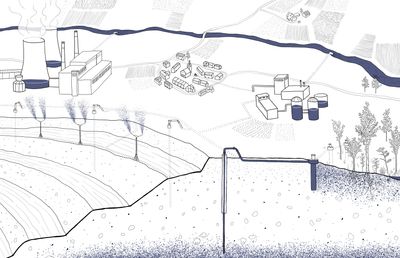The image appears to be a detailed, hand-drawn, black-and-white diagram, resembling a small-scale map or cartoon of an industrial area, possibly a nuclear plant or a mining operation. The background is mostly white, with various distinct features throughout. On the left side of the image, there are large buildings and two prominent vertical towers with smoke billowing out, suggesting a factory or industrial complex. Directly to the right, there is a cluster of smaller buildings that could be homes or additional facilities. Further to the right, even larger buildings and silos can be seen, potentially part of the industrial site. 

Behind these structures, a blue line stretches horizontally across the top of the image, which might represent a river or a road. Adjacent to the industrial section, and towards the far right, small shapes might indicate trees or other types of vegetation. 

The bottom part of the drawing includes various shapes and lines, potentially pipes or underground infrastructure used for drilling or mining operations. There are two vertical shafts drawn into the ground, one deeper and centrally located, and another slightly to the right and shorter. The elevation of the ground decreases towards the left side of the image. In the foreground, some plants and additional small structures are visible, enhancing the complexity of the drawing. Despite the varied interpretations, the scene cohesively represents a blend of industrial and natural elements in a meticulous, illustrative style.